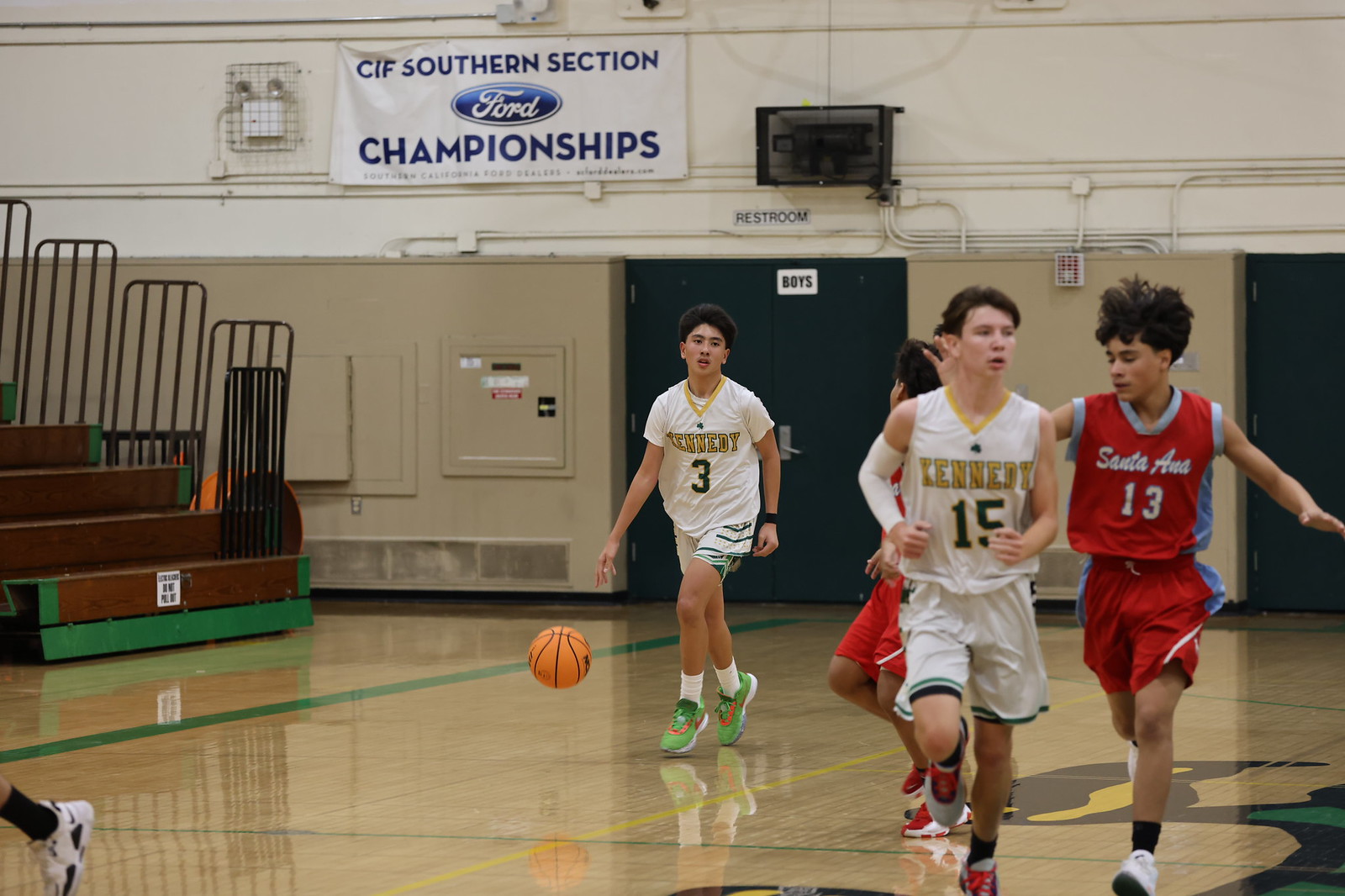This detailed photograph captures a high school basketball game taking place on an indoor court. The court floor is light brown with green, yellow, and black markings. In the image, four players are visible, with two wearing white uniforms that say "Kennedy" and two in red uniforms that say "Santa Ana." The players are mainly positioned on the right side of the image and appear to be running towards the camera, with the player farthest from the camera controlling an orange basketball. The indoor stadium features beige lower walls and white upper walls. On the upper wall, there is a prominent banner that reads "CIF Southern Section Championships," sponsored by Ford. The background includes blue double doors, another door towards the middle right, and pullout stands towards the middle left. A sign on a door says "Boys," likely indicating the locker room.